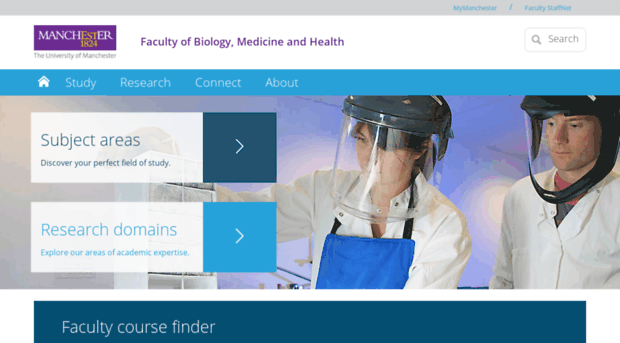The image depicts the website homepage of the "Faculty of Biology, Medicine, and Health" of the University of Manchester, originally established in 1824. The header features a prominent purple rectangle with the text "Manchester 1824" displayed horizontally. The word "Manchester" is in white, while "EST" and "1824" are highlighted in gold, adding a unique visual appeal. Directly beneath this, "The University of Manchester" is written in gray on a white banner. 

On the right side of the header, there's a search bar with a magnifying glass icon, and above it, a gray bar with the text "myManchester/faculty," indicating personalized access for users. Below the white banner, a blue navigation bar prominently displays links labeled "Study," "Research," "Connect," and "About."

The main section features a lab scene with a woman wearing a lab suit, helmet, and face guard, emphasizing the university’s focus on scientific research. Overlaid on this image are two rectangular buttons: the first one, labeled "Subject Areas: Discover Your Perfect Field of Study," and the second, "Search Domains: Explore Our Areas of Academic Expertise," both indicated with right arrows for further navigation. Beneath this, there's a banner titled "Faculty Course Finder," guiding users to explore available courses.